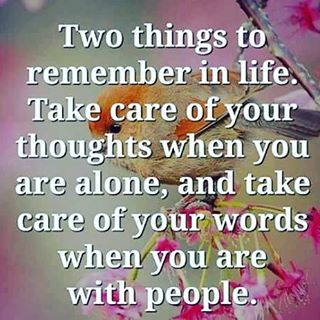This is an inspirational graphic image featuring a small bird with vividly colored plumage. The bird, possibly a finch, budgie, or swallow, has striking orange feathers on the top of its head, yellow on its body, and black tail feathers. It's perched on a tree branch adorned with light pink and bright pink flowers, hinting at a spring setting. The background consists of pastel pink and green hues, providing a serene atmosphere. Overlaid on the image in white text is a motivational message: "Two things to remember in life: Take care of your thoughts when you are alone, and take care of your words when you are with people." The textual advice makes the image not just a visual treat but also a source of sage wisdom, typically shared on social media platforms.